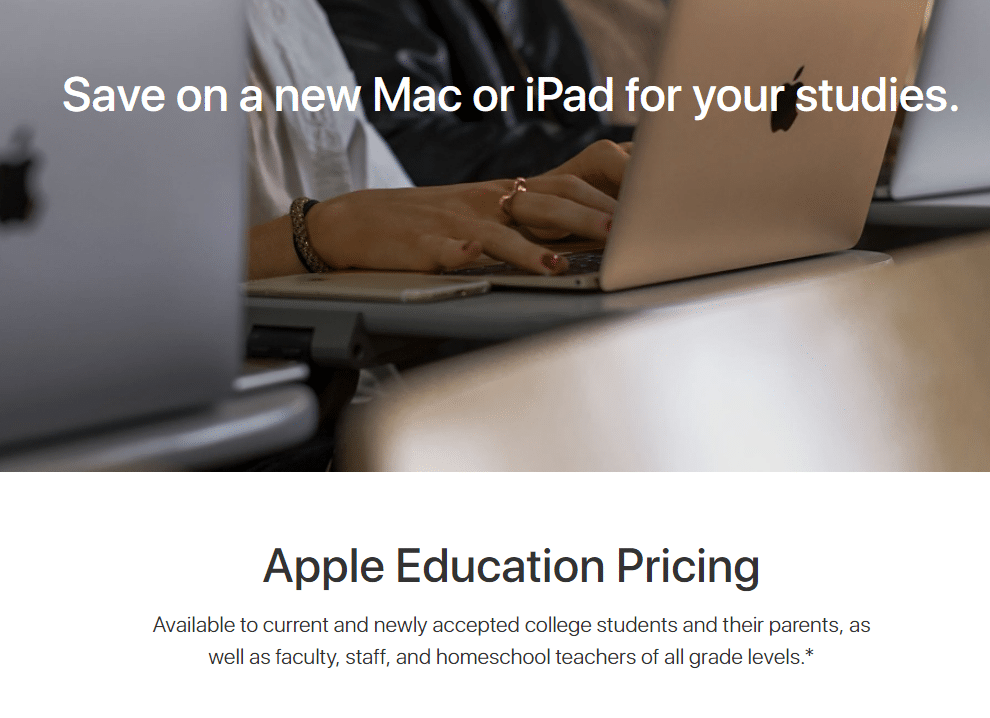This is a detailed caption for the image:

---

The advertisement from Apple is divided into two sections. The top section features an image of several students using Apple MacBooks in a study environment. The main focus is on a student working on a beige-colored MacBook, distinguishable by their rings, red-painted fingernails, and bracelets. This student's phone is also visible next to the MacBook. Surrounding this student, there are other students to the left and right with silver-colored Macs. The only visible parts of these students are their hands and their shirts, which are either black or white. The image is partly obscured by a blurred desk in the foreground, indicating the setting might be a classroom or study space. Superimposed on this image is white text that reads: "Save on a new Mac or iPad for your studies."

The bottom section of the ad contains black and white text. Prominently displayed in bold and large font is the headline: "Apple Education Pricing." Beneath this, a smaller subtitle provides additional details: "Available to current and newly accepted college students and their parents, as well as faculty, staff, and homeschool teachers of all grade levels."

---

This descriptive caption provides a clear and comprehensive depiction of the advertisement's visual layout and the information it conveys.